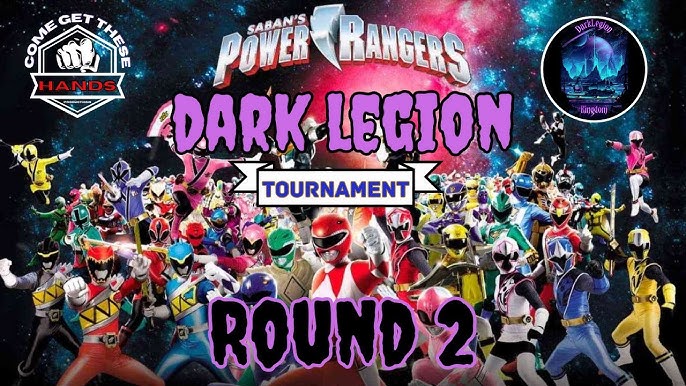The image is a detailed poster advertising "Saban's Power Rangers Dark Legion Tournament: Round Two." Dominating the center from top to bottom, bold white text reads "Saban's Power Rangers," with "Dark Legion" in vibrant purple beneath it. Below these, a white banner marked "Tournament" stands out, followed by "Round Two" at the bottom in black font trimmed with purple. The backdrop features a dynamic space scene blending red and blue hues.

At the upper left corner, in white font, a call to action reads "Come get these hands," accentuated by an icon of a fist. On the opposite top corner, a white circle contains the purple text "Dark Legion Kingdom," though the image inside the circle is difficult to decipher.

The poster showcases a multitude of Power Rangers, approximately 25 to 30, depicted in a kaleidoscope of colors including red, blue, yellow, green, purple, pink, and white, with a notable red Ranger centered prominently. The diverse array of Power Rangers outfits stands against the cosmic background, celebrating the vibrant spectrum of this iconic superhero team.